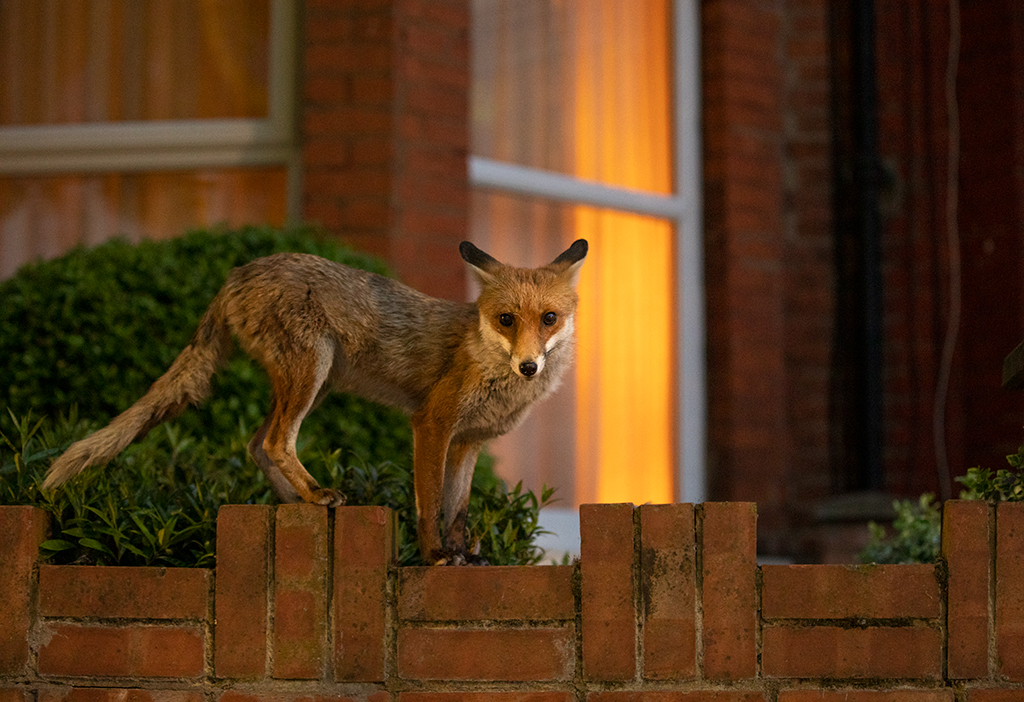In this detailed image, we see an outdoor scene captured possibly in the early evening. The photograph is rectangular, measuring approximately five to six inches wide and four inches high. Central to the image is a small, reddish-brown fox perched on a distinctive brick wall. The wall has a repeating pattern with two horizontally-laid bricks alternating with three vertically-aligned ones, creating an uneven surface. The fox is positioned with its front paws on the lower part of the wall and its back paws on the higher section, giving it a poised, attentive stance. 

The fox has striking features: black-tipped, slanted-back ears, a red face with a white underside that extends from its chin down to its neck, and pronounced red legs. Its back fur transitions to a brown shade, and it sports a thin, long brown tail. The animal’s large, dark eyes and pointed nose, which is dark with a white underside, add to its distinctive appearance. Behind the fox, there is a lush green shrub adding depth to the scene.

In the background, a brick house stands with bright amber light spilling from a window framed in white. The window's curtains are drawn, suggesting a cozy indoor space. Combined, these elements create a richly textured and atmospheric outdoor scene.